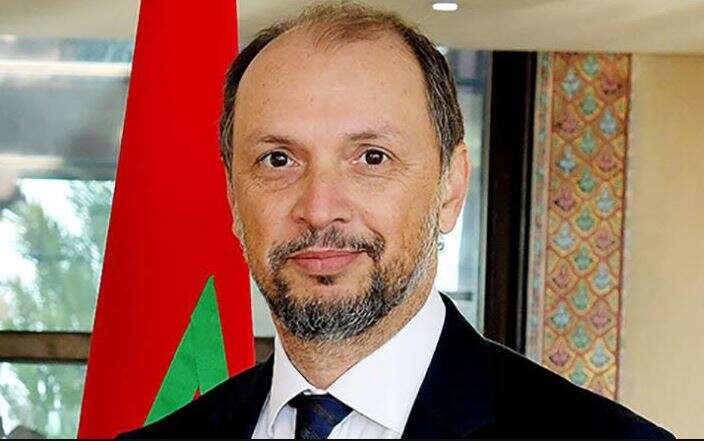This is a detailed photograph of an older man, likely in his late 50s or early 60s, captured from the shoulders up. He is dressed in a black suit with a white collared shirt and a blue tie. The man has a well-trimmed, salt-and-pepper beard and mustache, and his balding head features sparse hair on top but more on the sides. His dark brown eyes gaze directly at the camera, giving him a gentle and approachable demeanor. 

Behind him, the room is well-lit with a tan ceiling and a pot light visible above. To his right, you can see an ornate window frame in colors of yellow, blue, green, and burgundy, through which green foliage outside is visible. On the wall behind him, there is a vibrant, patterned wallpaper border in red, green, and blue on a yellow background. Additionally, a red flag with a green triangle sprouting from its bottom edge is prominently displayed over his right shoulder, adding depth and context to the scene.